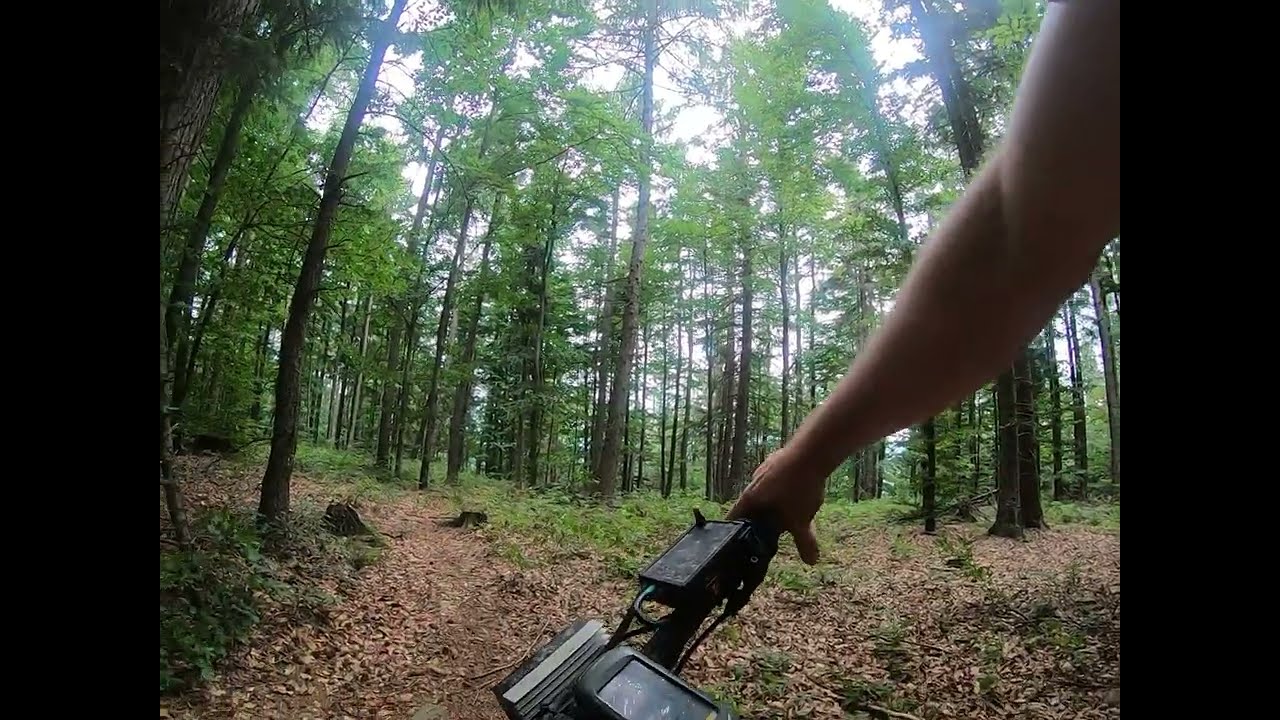The image is a horizontally rectangular, full-color photograph taken outdoors during the day, framed with a thick black border on the left and right. The scene unfolds in a tranquil forest, where tall, green-leaved trees stand under a hazy sky with sunlight filtering through the branches. The ground is blanketed with dead leaves, scattered rocks, and dirt, hinting at a well-trodden path veering slightly to the left.

In the foreground, a Caucasian person’s right arm, bare due to the warm weather, grips the black handlebars of a dirt bike or motorcycle, which is tilted to the left as if being set down carefully. The handlebars feature a couple of digital gauges or possibly a cell phone mount. The curved appearance of the trees near the edges suggests a fish-eye lens effect, adding a dynamic perspective to the serene setting. Despite the vibrant outdoor scene, no other animals or people are visible, enhancing the sense of solitude and peace.